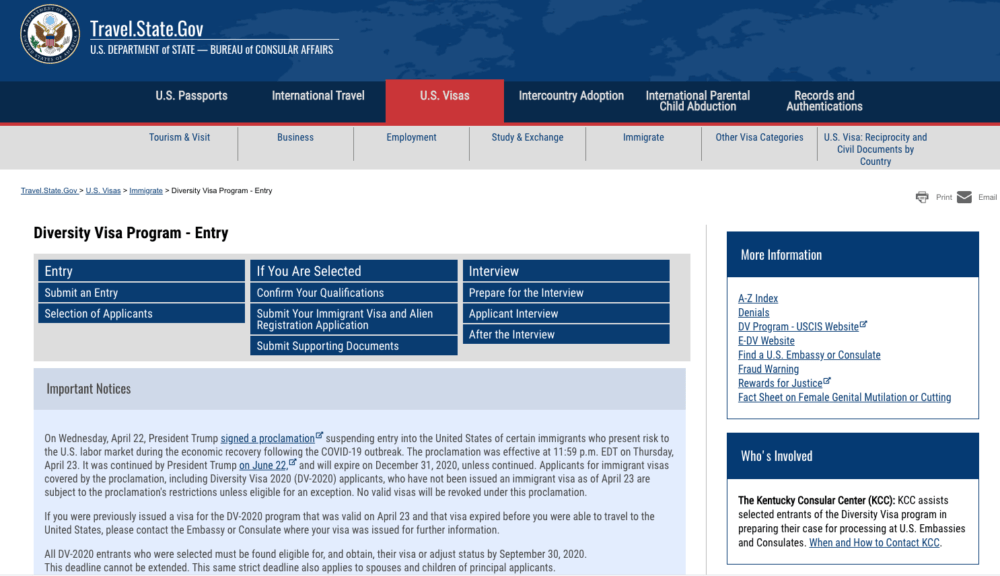The image is a screenshot from the travel website travel.state.gov, specifically the U.S. Department of State-Bureau of Consular Affairs section. At the top of the image, there is a navy rectangle featuring the text “U.S. Department of State - Bureau of Consular Affairs.” The word "Consular" is clarified phonetically as C-O-N-S-U-L-A-R. This navy rectangle appears to have subtle continent outlines embedded within it, blending shades of navy and lighter blue.

Beneath this header, a deeper navy rectangle displays several key topics related to travel and visas. These topics include "U.S. Passports," "International Travel," "U.S. Visas," "Inter-Country Adoption," "International Parental Child Abduction," and "Records and Authentication." The term "U.S. Visas" stands out prominently in red, highlighting its significance.

A horizontal line at the bottom of this deeper navy rectangle demarcates it from the lower part of the image. The lower section lists additional categories relevant to visa information and services, captioned as "Tourism and Visit," "Business," "Employment," "Study and Exchange," "Immigrate," "Other Visa Categories," and finally, "U.S. Visa, Reciprocity and Civil Documents by Country."

Overall, the structured layout and highlighted sections guide users through various aspects of international travel and visa services provided by the U.S. Department of State's Bureau of Consular Affairs.